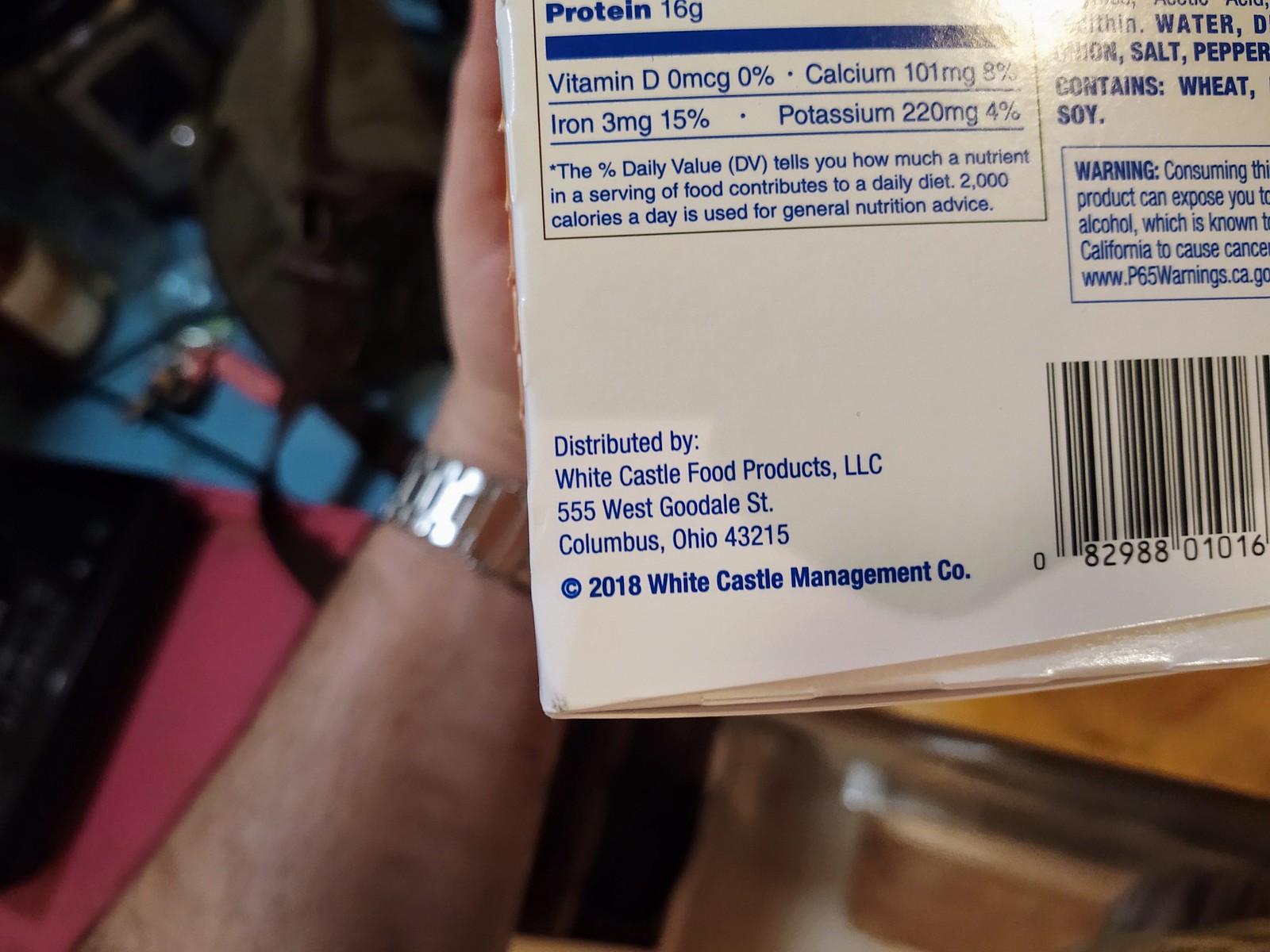The image depicts the backside of a white product box, believed to be associated with food items. At the bottom of the box, the text reads "Distributed by White Castle of Food Products LLC," followed by an address. There is also a copyright notice stating "2018 White Castle Management Co." To the right of this text, there is a barcode label.

In the top left corner of the box, the bottom section of the Nutrition Facts panel is visible. The readable portions indicate that the product contains 16 grams of protein, 0 mcg of Vitamin D (0% of the daily value), 101 mg of calcium (8% of the daily value), with listings for iron and potassium also present but not fully visible. 

To the right of the Nutrition Facts, the box lists the ingredients, along with a warning label below it. 

In the background, a hand holding the box is seen, wearing a silver watch. The floor is somewhat blurred but shows a scattered array of items including a backpack, a blue pad, a red pad, a black bag, and a black machine, all on a wooden floor. A table is positioned at the bottom right corner of the image.